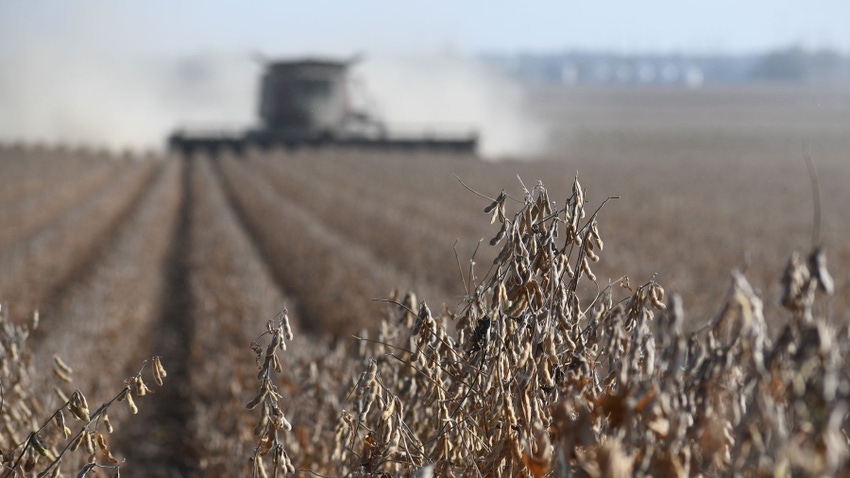The photograph captures a rural landscape during the day, showcasing an expansive field under a clear blue sky. The main focus is on the foreground, where a cluster of dried, brown, and wrinkled plants stands in sharp detail. Their thin, gray stems are adorned with tan seed-like pods, indicative of severe dehydration possibly due to a prolonged drought. In the blurred background, a large harvester machine is plowing the field, emitting clouds of gray dust on either side as it maneuvers. Though out of focus, the harvester’s distinct rectangular harvesting blade is noticeable. To the top right, faint grayish forms, potentially distant buildings, are just visible, adding depth to the pastoral scene.